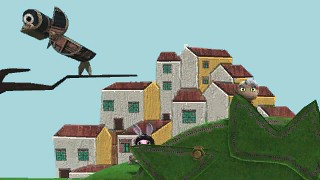The image showcases a vibrant 3D scene under a clear blue sky. In the background, a collection of eight uniquely designed houses is visible, each characterized by white walls, red rooftops, and teal-green windows, evoking styles ranging from Mediterranean to bungalow architecture. The foreground features a lush grassy field interspersed with grass hedges patterned with zipper-like designs. On the middle right of the image, a puppet with a brown head and a doctor's hat stands prominently. Meanwhile, the bottom left corner reveals a playful rabbit, distinguishable by its two ears and ninja costume. In the upper left area of the scene, a single tree branch extends outward, intriguingly adorned with two or three treasure chest-like objects with metal rims. The overall size of the picture is relatively modest.